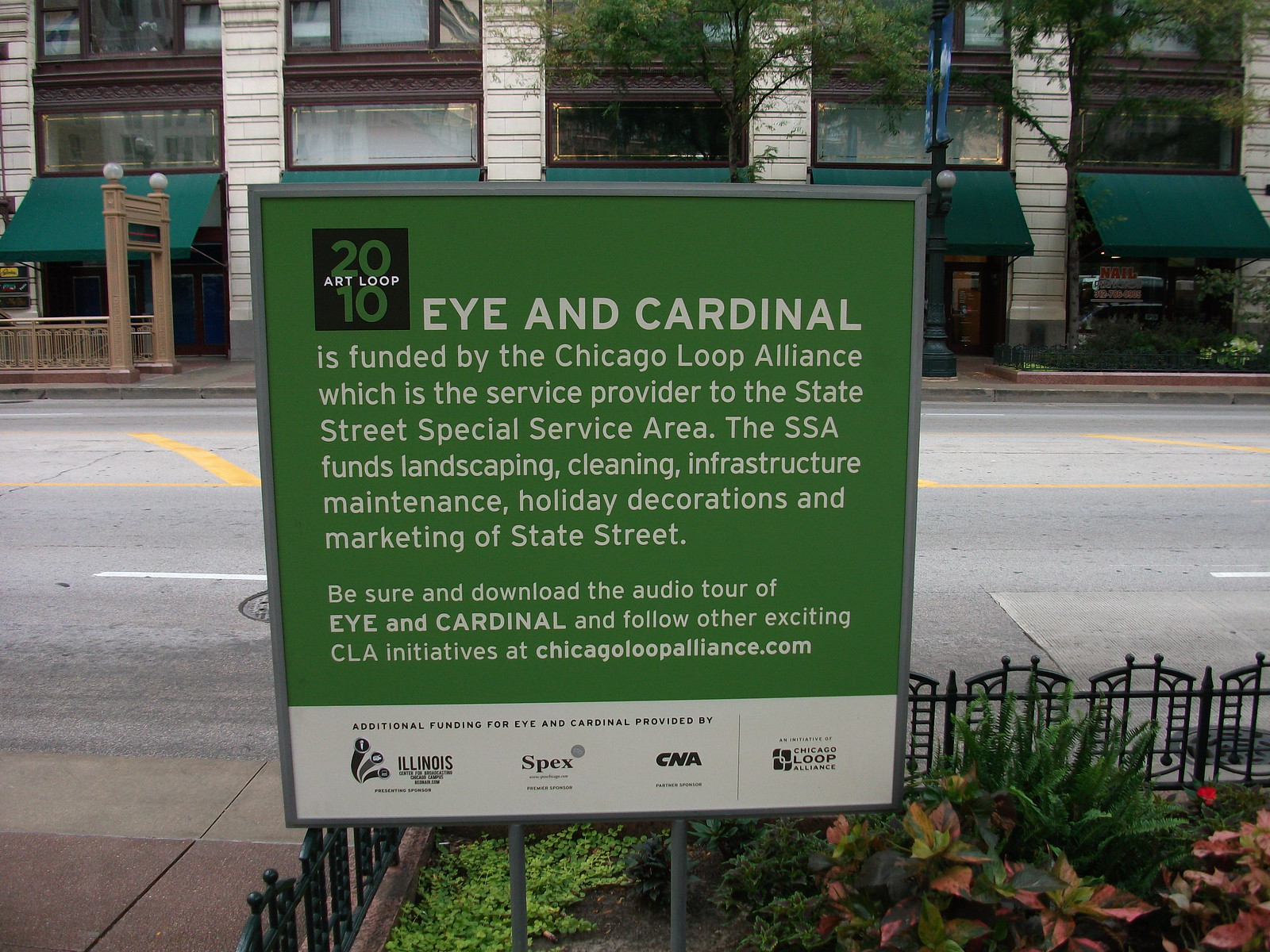This photograph captures a sign situated in a small flower garden along a sidewalk. The sign, bordered by a steel frame and supported by two metal poles, stands prominently in the foreground. It features a green background with white text and is partially framed by a small metal fence enclosing the garden, complete with shrubbery and small bushes.

At the top left of the sign is a black square logo, marked with "2010 Art Loop" in green and white lettering. The main text on the sign reads: "I and Cardinal is funded by the Chicago Loop Alliance, which is the service provider to the State Street Special Service Area (SSA). The SSA funds landscaping, cleaning, infrastructure, maintenance, holiday decorations, and marketing of State Street. Be sure to download the audio tour of I and Cardinal and follow other exciting CLA initiatives at chicagoloopalliance.com."

Below this main text is a white section listing additional funding contributors, adorned with logos from various organizations, including Illinois, Spex, CNA, and the Chicago Loop Alliance.

In the background, a plain asphalt street with blue and white lines is visible, along with a sidewalk and a building adorned with dark green awnings. To the left, the entrance to a subway, marked by a small tower and brown fencing, adds to the urban landscape.